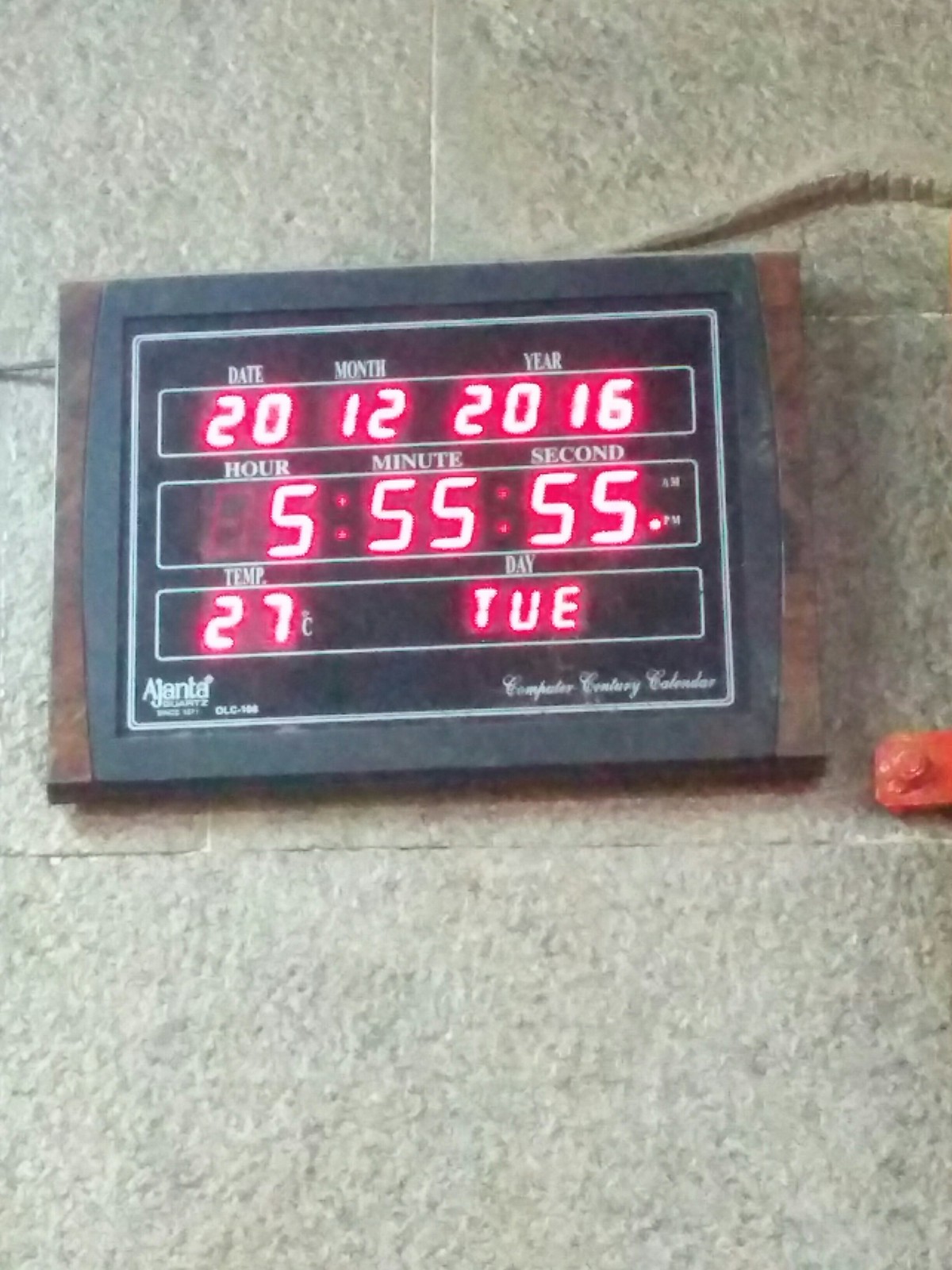The image captures a rectangular LED panel displaying an array of information including date, time, temperature, and the day of the week. The display indicates that it is the 20th of December, 2016, and the current time is 5:55. The temperature is shown as 27 degrees Celsius, and the day is Tuesday. The panel, which features the logo of a company named Aljanta in the bottom left corner, is made of plastic with slightly rounded edges and is mounted on a stone wall. Below the panel, there is a red object resembling a bolt also affixed to the wall. The LED panel, which stands for light-emitting diode, serves as a multifunctional digital display.